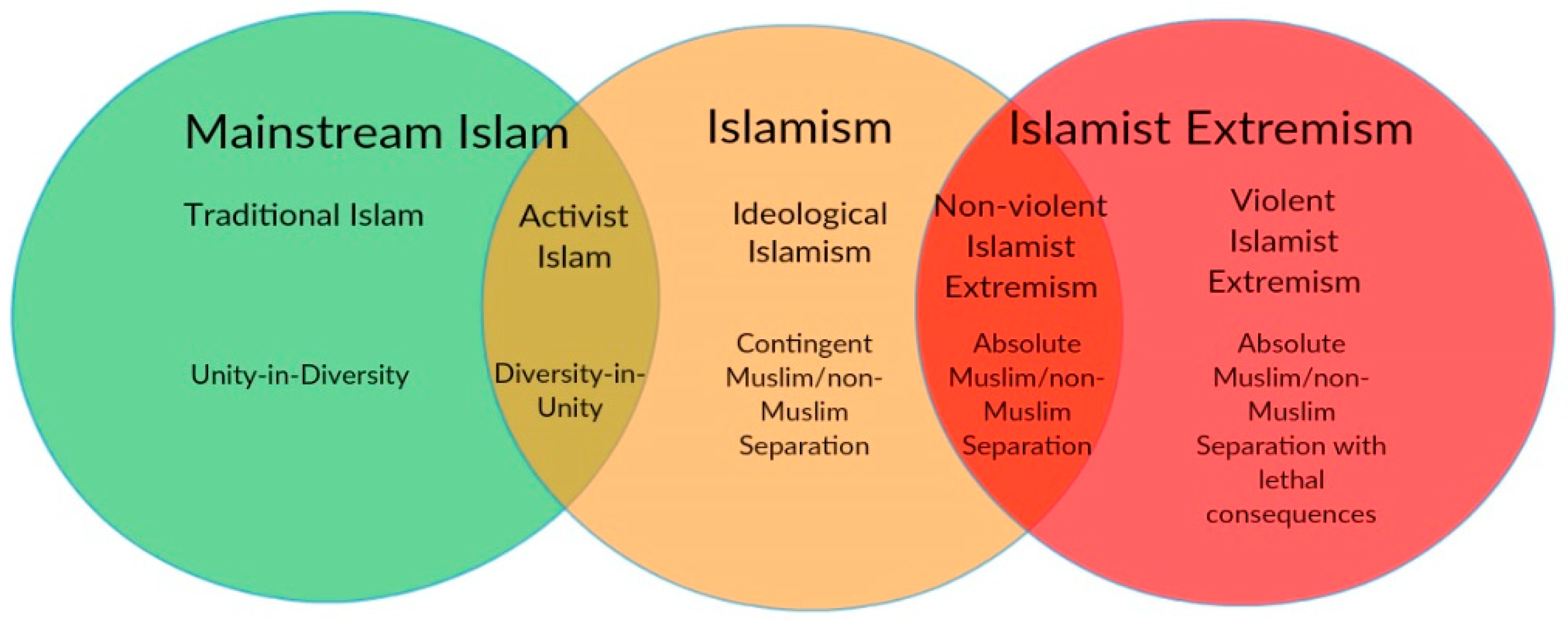The horizontally rectangular digital image presents a detailed explanation of different perspectives within Islam through three overlapping circles, each bordered faintly in blue against a white background. The leftmost green circle is labeled "Mainstream Islam," including subcategories "Traditional Islam" and "Activist Islam," and emphasizes the phrases "Unity in Diversity" and "Diversity in Unity." Next, the orange middle circle is labeled "Islamism," with subcategories "Ideological Islamism," and it discusses "Contingent Muslim-Non-Muslim Separation." Fascinatingly, this orange circle overlaps with the green circle, indicating areas of shared concepts. The right-most red circle is divided further: one section labeled "Non-Violent Islamist Extremism," mentioning "Absolute Muslim-Non-Muslim Separation," and another section denoting "Violent Islamist Extremism," which emphasizes "Absolute Muslim-Non-Muslim Separation with Lethal Consequences." This overlapping design illustrates the nuanced distinctions and connections between various interpretations and extremities within Islam.